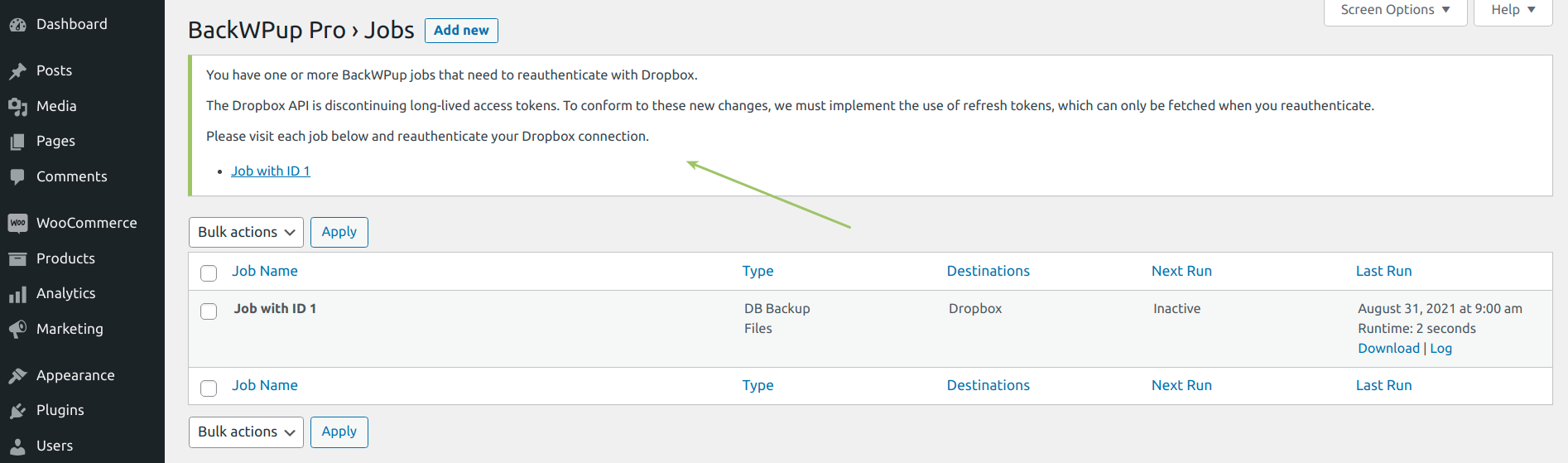The image showcases a website with a detailed interface. On the left sidebar, it features a black rectangle with the word "Dashboard" in white text at the top, accompanied by a gauge icon. Below it, there are various icons and labels: a pin icon next to "Posts," a camera and music note next to "Media," two rectangles labeled "Pages," and a text box labeled "Comments." Following that, there’s a message bubble icon with the word "Woo" and below it "WooCommerce." Next, a filing cabinet icon with "Products," followed by a bar graph icon for "Analytics," a megaphone icon labeled "Marketing," a paintbrush icon for "Appearance," a plug icon for "Plugins," and lastly, a person icon for "Users."

The main content section of the website has a light gray background. At the top, it says "BackWPup Pro" with an arrow pointing right towards a label "Jobs." There is a blue notification reading, "You have one or more BackWPup jobs that need to reauthenticate with Dropbox. The Dropbox API is discontinuing long-lived access tokens. To conform to these new changes, we must implement the use of refresh tokens, which can only be fetched when you reauthenticate. Please visit each job and reauthenticate your Dropbox connection." This notification is highlighted by a green arrow.

Below this message, another section in blue text outlines the job details, labeled "Job Name," "Type," "Destinations," "Next Run," and "Last Run," all encased in a white rectangle. Further descriptions of individual jobs are listed underneath.